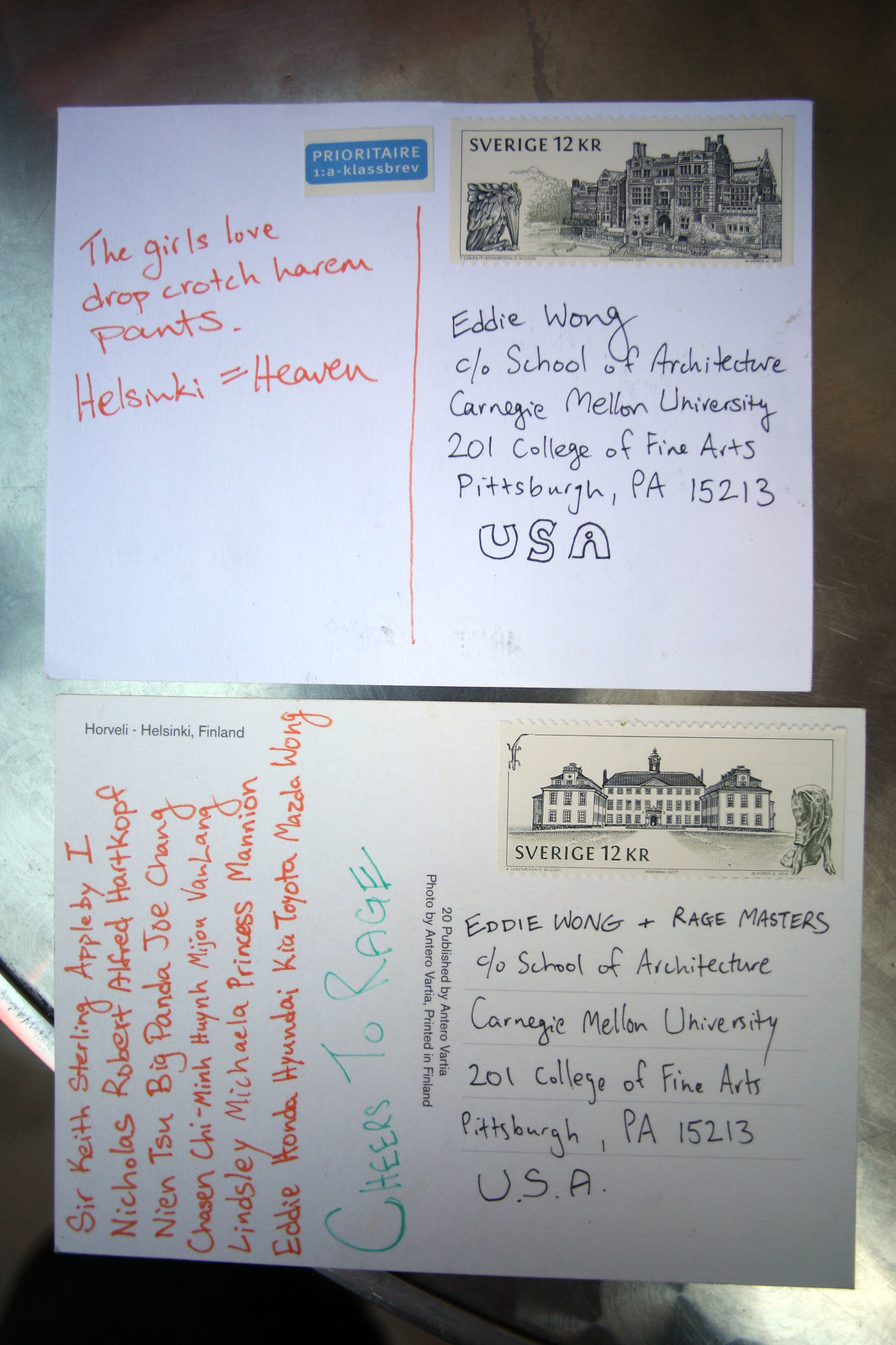The image is a color photograph in portrait orientation, featuring two postcards stacked vertically, filling most of the frame. Both postcards are addressed to Eddie Wong, with detailed handwriting specifying the School of Architecture at Carnegie Mellon University, 201 College of Fine Arts, Pittsburgh, PA 15213, USA. 

The top postcard appears newer, with a white background. It has a vertical red line marking a separation on the left and a rectangular stamp in the upper right corner. The stamp, marked "SVERIGE 12 KR," features an intricate illustration of a raven and a large stone building. Above the address, in red ink, there is a note saying, "The girls love drop crotch harem pants. Helsinki equals heaven." A small sticker above this text reads "PRIORITAIRE 1 AC LOSPREV."

The bottom postcard is slightly older and darker in color. It too bears a "SVERIGE 12 KR" stamp in the upper right, displaying an image of a school. In the center, a vertical stamp reads "20 published by Ontero Varsha, photo by Ontero Varsha printed in Finland." The top left corner has "Horvelli - Helsinki, Finland" printed in black ink. Written vertically in red ink on the left side are multiple names, including "Sir Keith Sterling Appleby 1, Nicholas Robert Alfred Hartkoff, Nien Su Big Panda Joe Chang, Chasen Chimin Hyun Miju Van Lang, Lindsey Michaela Princess Mannion, Eddie Honda Hyundai, Kia Toyota Mazda Wong," and in green ink, "Cheers to Rage." 

Both postcards capture a sense of personal messaging and artistic postal elements with stamps and scribbled notes enriching their surfaces.